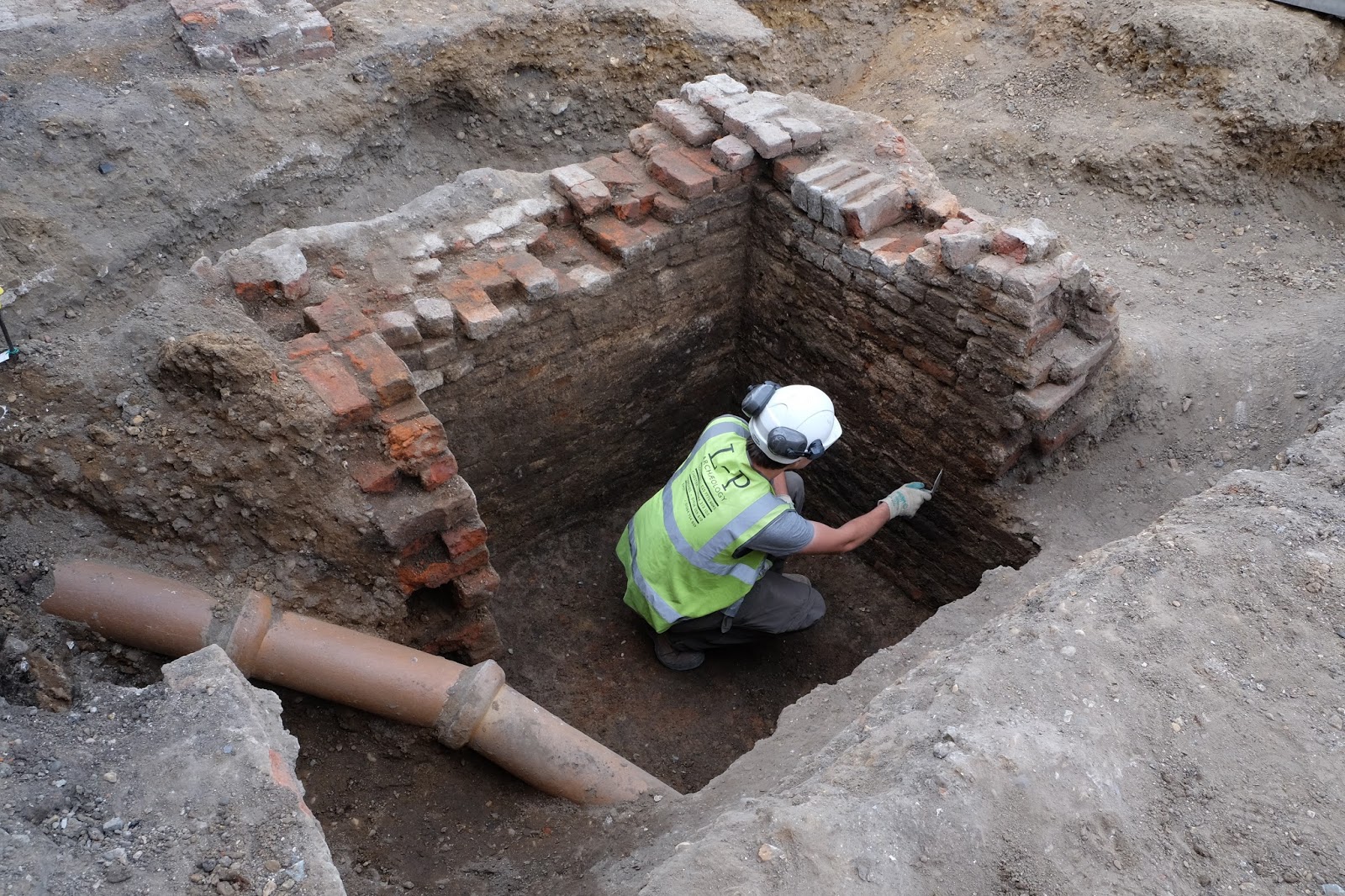In the center of the image, a man is kneeling down in a shallow, rectangular pit, approximately five to six feet deep. He appears to be engaged in excavation work, possibly as part of an archaeological or geological preservation project. The pit is surrounded by old red brick walls, with loose gravel and soil scattered around the top right and left corners. 

The man is dressed in a neon green high visibility safety vest with reflective gray bars and black lettering on the back that reads "L-P archaeology." He is also wearing a white safety helmet equipped with ear protection, which is flipped up towards the back of the helmet. His attire includes a short-sleeved gray shirt, gray pants, brown gloves, and gray boots. 

The man is using a shovel-like scalpel tool to scrape at the brick wall on his left, suggesting that he is carefully uncovering or cleaning the brick surface. To his left, a red clay pipe extends into the pit, indicating the possible presence of an old sewage or foundation system. The setting is characterized by the contrast of red bricks, gray soil, and the man's brightly colored safety gear, highlighting his meticulous work in this small, exposed area.